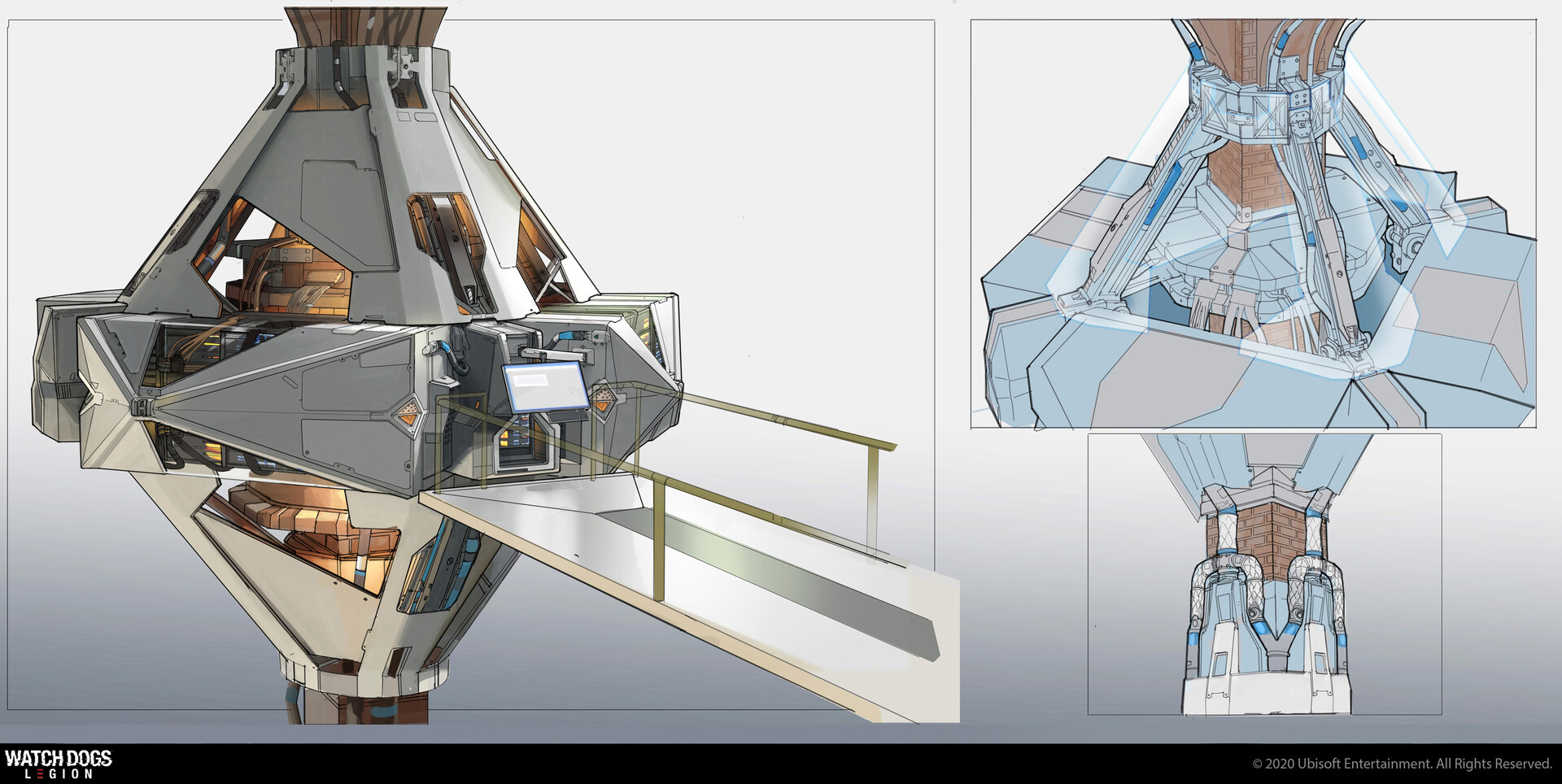The image is a widescreen landscape, predominantly showcasing a large, futuristic spaceship or space station. The craft, with a conical design, has a wider middle band that tapers towards the top and bottom, featuring a grey upper half and a white lower half. On its front, a gangway platform extends downwards to the bottom right, characterized by a white surface with a shiny green and silver strip down the center, flanked by golden-bronze handrails. Inside, the spacecraft displays a complex array of glass panels, coils, and copper-like machinery resembling large magnets, with a computer interface and computing storage system at the top of the gangway.

Additionally, to the right side of the image, a blue and beige cross-sectional diagram of the same spacecraft or space station is depicted, providing a top-down view and revealing an inner structure that includes a bronze core resembling a brick chimney. Along the bottom of the image is a black strip containing a white text on the left that reads "Watch Dogs Legion" with a smaller, less legible text beneath it stating the copyright by 2020 Ubisoft Entertainment. Similarly, on the right side of the black strip, there is more white text that is greyed out and difficult to read. This highly detailed image appears to be a mock-up from a futuristic video game environment, likely indicating a space station or a bridge within a futuristic factory.